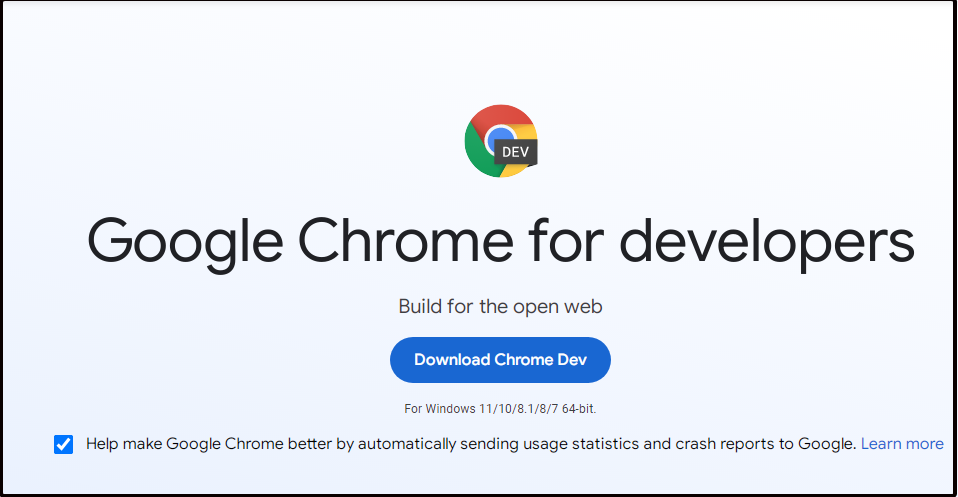The image depicts a webpage viewed on Google Chrome, characterized by a predominantly light blue, almost white, background. At the top of the page, there is a prominent Chrome logo, accompanied by a small black box with the word "DEV" in white, signifying the developer version. Below this header, bold black text reads "Google Chrome for developers," followed by a smaller black text slogan, "Build for the open web."

Positioned underneath these descriptions, a blue button with white text invites the user to "Download Chrome Dev." Directly below this button, there's a note in diminutive black print stating compatibility with various Windows versions: "Windows 11/10/8.1/8/7 64-bit."

Towards the bottom left of the page, there is a blue box containing a white checkmark. Adjacent to this icon, black text encourages users to "Help make Google Chrome better by automatically sending usage statistics and crash reports to Google," with an accompanying blue "Learn more" link for additional information.